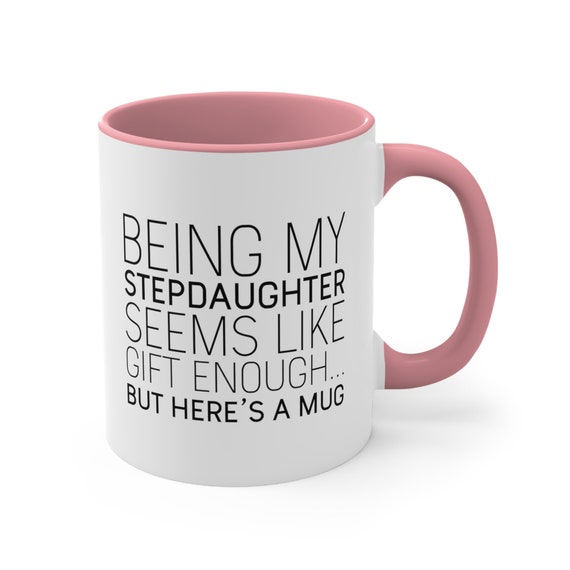This image features a tall, white coffee mug with a matching pink handle on its right side, and a pink interior and rim. The mug stands alone against a pure white, borderless background, giving it a CGI-like appearance due to the flat lighting. The mug bears a bold, black text in all caps, with varying font weights: "BEING MY" at the top followed by a shorter, bolder "STEPDAUGHTER," then "SEEMS LIKE" in a similar style to "BEING MY," "GIFT ENOUGH" in a slightly lighter font, and finally, "BUT HERE'S A MUG" at the bottom in an even bolder text, ending with a dot, dot, dot. The phrase seems to indicate the mug is a humorous gift from a step-parent to their stepdaughter.